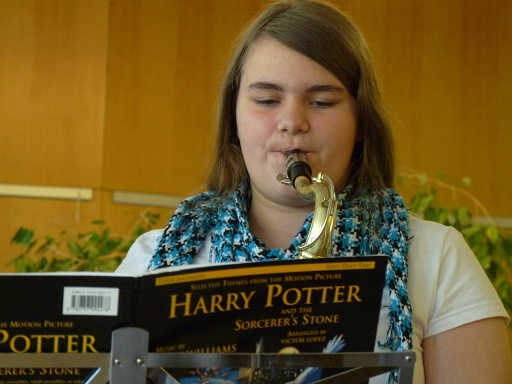In this detailed image, we see a young girl, possibly in high school, with shoulder-length, dark blonde to brown hair parted to the side. She is light-skinned and dressed in a white short-sleeved t-shirt paired with a blue-black patterned scarf around her neck. She is playing a saxophone, with the gold mouthpiece visible between her lips. Resting on a silvery music stand in front of her is an open book for music sheets, titled "Selected Themes from the Motion Picture Harry Potter and the Sorcerer's Stone". The book has a distinct black and yellow cover with a white and black barcode on the back. She appears deeply focused on the music. In the background, there is a wooden wall adorned with green leaves and a golden-yellow curtain, creating a warm and slightly staged atmosphere.